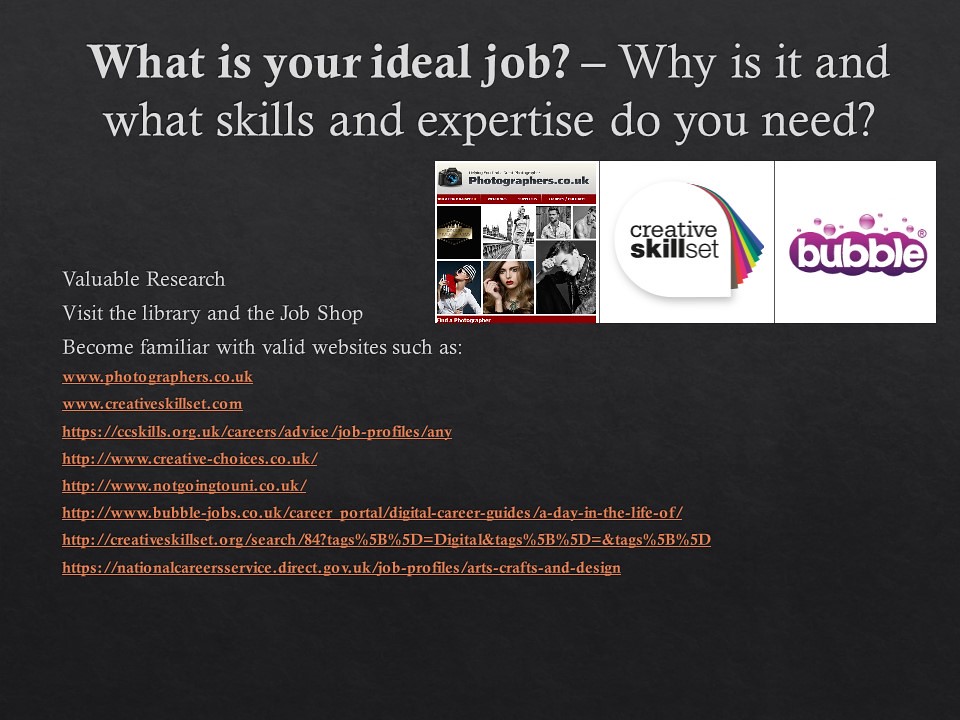The image depicts a rectangular, horizontal postcard, primarily with a black background. The prominent question, "What is your ideal job? Why is it and what skills and expertise do you need?" is written in bold white letters at the top, suggesting it might be an educational prompt used in classrooms to engage students in career planning. The postcard encourages valuable research, urging viewers to visit the library, the job shop, and become familiar with reputable websites. A series of websites is listed in orange text, occupying a significant portion of the image, including www.photographers.co.uk, www.creativeskillset.com, https://ccskills.org.uk, https://careers.com, https://advice.com, and others. On the right-hand side, there are a few photographs and purple "Bubble" graphics, also pointing towards resources like Creative Skillset. The varied colors—white, blue, red, orange, green, yellow, and purple—add visual interest. This curated collection of resources and visuals appears designed to guide individuals in identifying and pursuing their ideal careers, particularly in creative fields.